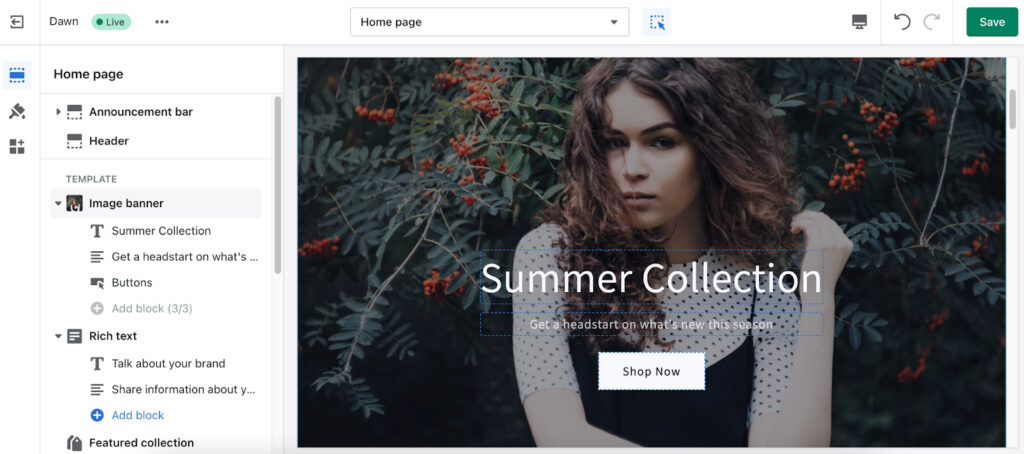On this page, there is a white background with light gray lines along the side and at the top. On the top line, there is a small empty box with a left-pointing arrow. Next to it is a small blue box followed by an icon that looks like a paintbrush. There are also three small squares with a placeholder for a fourth square which contains a plus symbol. A light vertical line divides the space and the word "Dawn" appears next to it. Next, there is a small blue box containing a green dot along with the word "Live" and three small dots. Below this section, it displays "Home Page" and a small box labeled "Announcement Bar and Header." The word "Template" follows, with several subsections listed underneath it including "Rich Text" and "Featured Collection." A gray scroll bar runs down the side of the page.

Beneath that, there is an image with a dark background showcasing a large holly tree adorned with red berries. In the foreground stands a pretty girl with long, dark, curly hair, wearing a black and white polka dot shirt under a black top. In white text, it says "Summer Collection," accompanied by the phrase "Get a head start on what's new this season." Below this text, there is a white button with a gray "Shop Now" inscription.